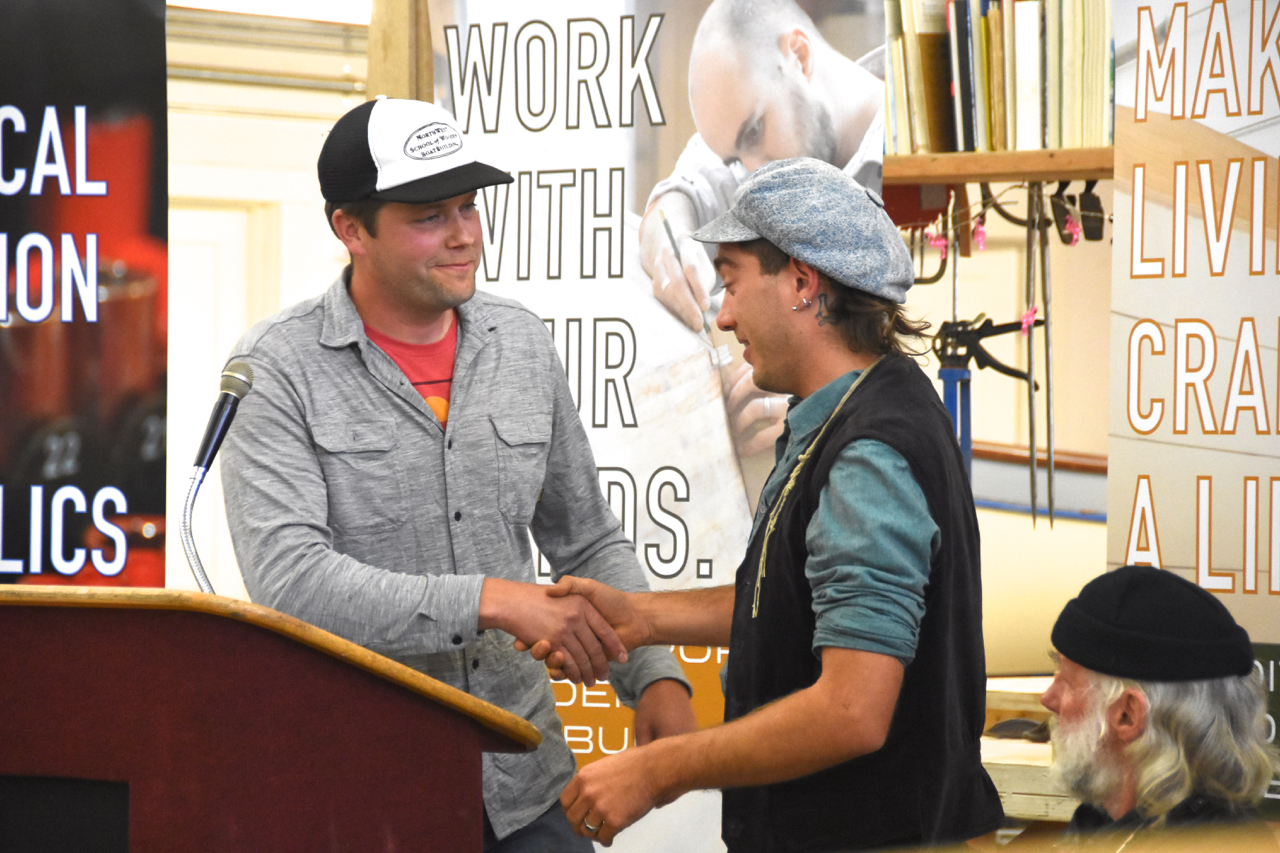In this detailed convention photograph, we see two men shaking hands in what appears to be a meeting room adorned with informational display boards and machinery. The man on the left is wearing a black and white trucker hat, a gray long-sleeved jacket with pockets, and a red t-shirt underneath. He stands behind a brown podium equipped with a microphone. The man on the right, who has medium-length brown hair, a gray hat, piercings, a tattoo behind his ear, and earrings, is dressed in a gray vest over a blue shirt. 

To the bottom right of the frame, an older man with long wavy gray hair and a matching beard is seated, wearing a black beanie. The background showcases three posters: one black with red details, another white with partially visible text reading "work with your hands," and a final one with discernible letters "C-M-A-K" and "C-R-A-A-L-I," as well as various images and tools. The scene captures a casual yet engaging moment likely related to some form of union or trade meeting.